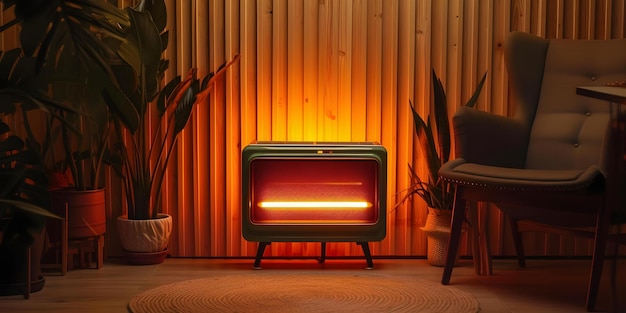The image depicts a stylized seating area, possibly a living room, with a strong retro aesthetic. At the center is a space heater, rectangular in shape with rounded edges, reminiscent of an old-fashioned TV. This heater stands on three diagonally outward-pointing legs. A glowing orange bar radiates light from its center, casting an ambient glow that highlights an array of surrounding potted plants. To the right of the heater, there is a leafy plant in a milk jug-shaped container that appears to be ceramic or plastic. On the left, a trio of plants is situated in varied pots: a white bowl-shaped pot containing a plant with long stems and large leaves, an orange cylindrical pot (possibly just lit to appear orange) with another tall-stemmed plant, and a traditional brown pot holding a fern-like plant.

Additionally, the setting includes a blue chair with armrests, slightly reclined, suggesting comfort and relaxation. This chair exhibits a 70s style with a fold indicating a footrest on its end. The room’s flooring is light wood, on which a circular woven carpet with concentric rings lies central. The back wall, orange and metallic, has a texture resembling a shipping container. Despite the room's dim lighting, the radiant orange glow from the heater provides sufficient illumination, creating a warm and inviting atmosphere.